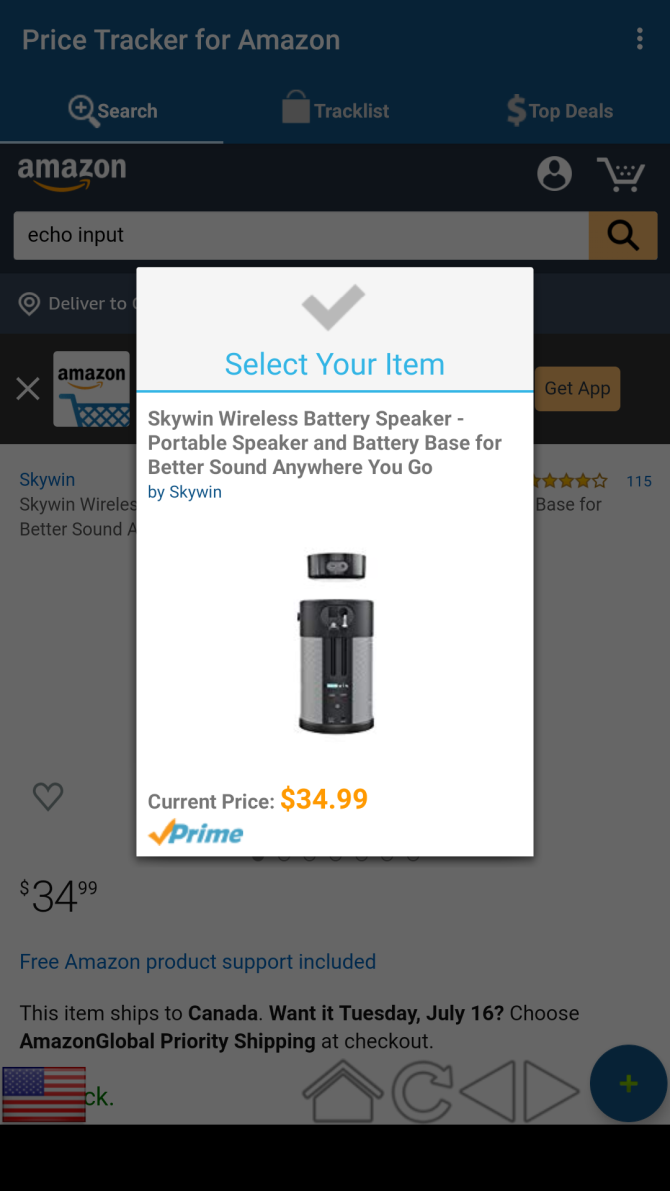The image is a screenshot from the mobile version of Amazon's shopping app, featuring a pop-up detailing a product. The pop-up, with a white and light gray background and a gray checkmark, prominently displays the Prime logo. In blue text, it prompts the user to "select your item." It highlights the "Skywind Wireless Battery Speaker," described as a portable speaker and battery base that enhances sound quality on the go. The product is priced at $34.99 and includes another Prime logo at the bottom left corner of the pop-up.

This pop-up partially obscures the underlying page, which has a blue-bordered header with white font reading "Price Tracker for Amazon." The header includes tabs for "Search," "Track List," and "Top Deals." In the search bar of this Amazon page, the term "echo input" is visible. Despite the pop-up, the bottom section of the page reveals text stating, "Free Amazon product support included." It also specifies that the item ships to Canada on Tuesday, July 16th, with the option to choose Amazon Global Priority Shipping at checkout. The interface includes an American flag icon, a home icon, refresh and navigation buttons, and a blue circle featuring a green plus sign at the bottom of the screen.